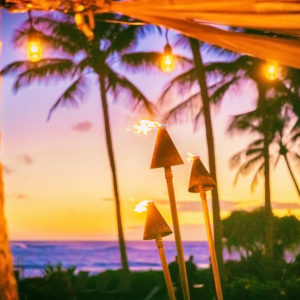The image, which appears blurry overall and square in shape, depicts an outdoor scene that resembles a Hawaiian luau, possibly at sunset. The centerpiece of the foreground features traditional Tahitian or Hawaiian tiki torches, each with a cone-like top and flames emanating from the tips. Above these torches, there are café-style lighting bulbs hanging from a brown platform, illuminating the scene with a warm yellow glow from at least three lights. The blurred background reveals tall palm trees, at least three or four, along with shorter ones, and lush green bushes. The sky is a blend of white, yellow, and purple hues, indicating a sunset over the ocean, which mirrors these colors. The ocean itself is visible with distinct blue waves, adding to the serene, tropical atmosphere.